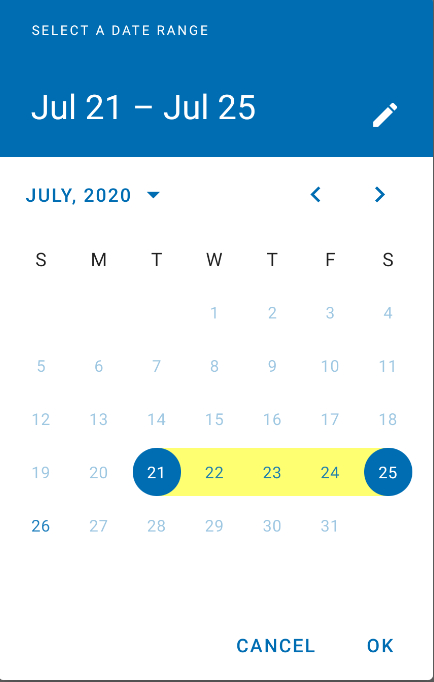**Descriptive Caption:**

Under the category of websites, the image presents a detailed view of an interactive calendar interface. At the top, a blue bar prominently displays the text "July 21st - July 25th" in white letters, with an option to edit this date range. Directly below, the header "July 2020" appears in blue letters on a white background. Navigation arrows are situated on either side, allowing users to move back to June or forward to August.

The calendar interface highlights the dates 21st and 25th in blue, while the dates 22nd, 23rd, and 24th are marked in yellow, indicating a continuous selection from the 21st to the 25th. At the bottom of the interface, options to "Cancel" or "Okay" provide the functionality to either accept or reject the chosen dates.

The calendar layout indicates that July 2020 starts on a Wednesday (the 1st) and ends on a Friday (the 31st). The days of the week, represented by the letters SMTWTFS, are displayed in black, while the majority of the calendar dates are shown in a very light bluish-gray. Notably, the 26th is highlighted in a brighter blue, suggesting a scheduled event on that day. This image captures the simplicity and functionality of a basic calendar interface with specific date selections highlighted.